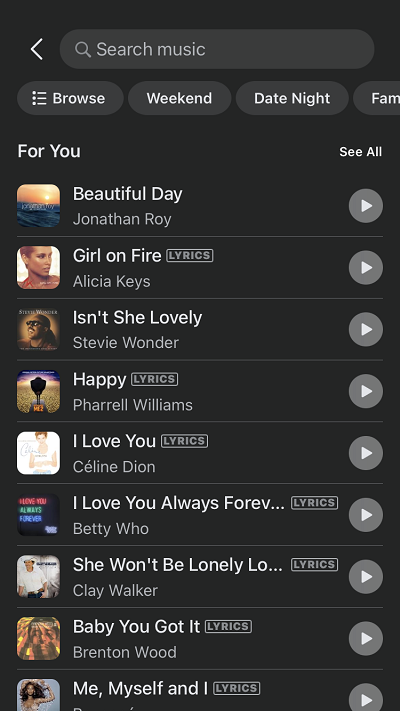Black background screenshot featuring a music browsing interface. At the top, there's a left-facing arrow next to a search bar with a magnifying glass icon, followed by category tabs: Browse, Weekend, Date Night, and For You. A "See All" option is also available.

The central section displays a list of songs, each accompanied by a right-facing circle with an arrow inside, indicating more options. The listed songs include:

- "Beautiful Day" by Jonathan Rory
- "Girl on Fire" by Alicia Keys, with a prominent "Lyrics" label in a rectangle
- "Isn't She Lovely" by Stevie Wonder, also with a "Lyrics" label
- "Happy" by Pharrell Williams, featuring a "Lyrics" label
- "I Love You" by Celine Dion
- "I Love You Always Forever" by Betty Who, abbreviated as "I Love You Always... f-o-r-e-v..."
- "She Won't Be Lonely Long" by Clay Walker, abbreviated as "She Won't Be L-o..."
- "Baby You Got It" by Brenton Wood
- "Me, Myself, and I" by Beyoncé (partially cut off)

The captions provide clear song titles, artists, and indicate which songs have lyrics available in a distinct rectangular label.